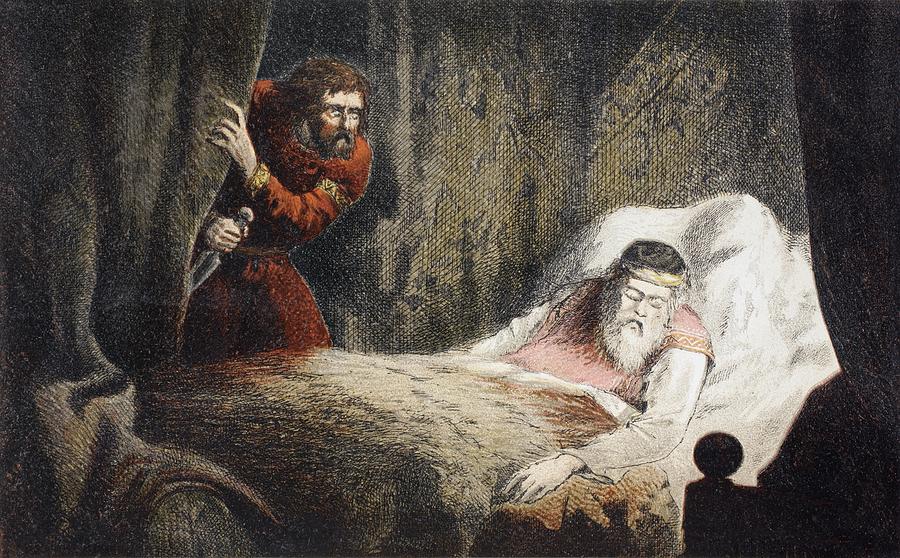This detailed image is a historical-style drawing, possibly done with pencil. It depicts a dramatic scene in a darkened bedroom where an old man, presumably a king due to the golden circle on his head, is sleeping in a grand canopy bed draped with dark curtains. The king, distinguished by his pale complexion and white beard, is dressed in a red nightshirt over a white long sleeve shirt, and is covered by a fur blanket. He lies on his left shoulder with his head tilted to the right and hands resting at his sides. Emerging from the left side of the image, partially concealed by the curtain, is an assassin with long red hair and a beard, dressed in a red outfit adorned with gold accents. The assassin is holding a knife in one hand and pulling back the curtain with the other, poised to approach the sleeping king. The intense atmosphere of the drawing is further highlighted by the contrast between the dormant king under the warm blanket and the impending danger represented by the stealthy, armed intruder.